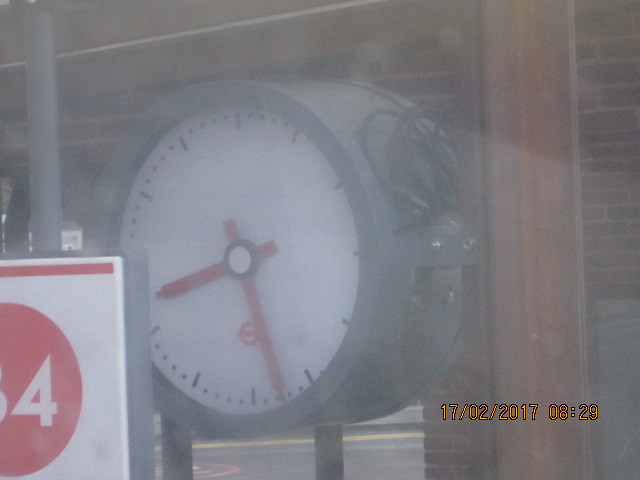In the image, the central focus is on a round clock with red arms. The minute hand is positioned between the 5 and 6, while the hour hand rests between the 8 and 9. A white dot holds the hands at the center of the clock face, which features dash marks indicating the hours. The clock is encased in a silver frame. To the bottom right, there is a digital display that reads "17-13-5-5-5" and "08:29." The right side of the image is cluttered with numerous cables, secured by bolts. The background shows a brick wall, adding a rustic element to the scene. In the bottom left corner, a white square with a red circle and partially visible white text, including the number "4," is noticeable. A silver pillar or pole is present to the left of the clock.